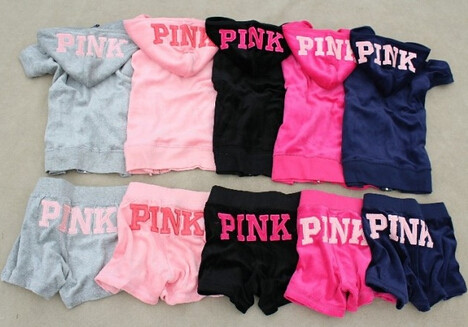The image depicts five sets of clothing that are likely designed for a very young girl, possibly around three or four years old, given their size. Each set consists of a short-sleeve, hooded top and matching shorts, all emblazoned with the brand name "Pink." The word "Pink" is prominently displayed on the hoodie of the tops and on the back of the shorts. The color palette includes a variety of shades: baby blue, light pink, black, a vibrant Barbie-pink, and a dark navy blue. Each outfit offers different hues and placements of the word "Pink," creating a diverse yet cohesive collection of small-sized attire.